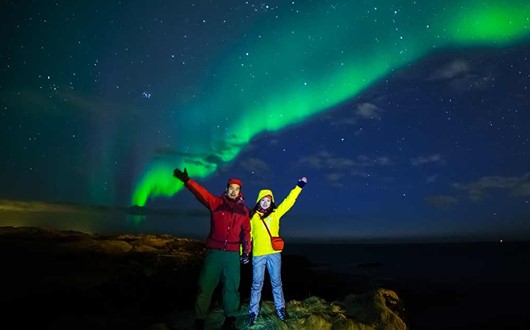A couple stands triumphantly on a mountaintop, high above sea level, beneath a stunning display of the Northern Lights. The woman, dressed in a yellow jacket with a red crossbody pocketbook and jeans, raises her left arm. The man beside her, clad in a red jacket, matching red scarf and hat, with green pants, mirrors her pose with his right arm. Together, their outstretched arms form a V shape. Behind them, a spectacular neon strip of the aurora borealis originates beyond the water and arcs magnificently across the clear, blue sky filled with scattered clouds. Below them, the sea stretches out, providing a vast, serene backdrop to this magical moment.